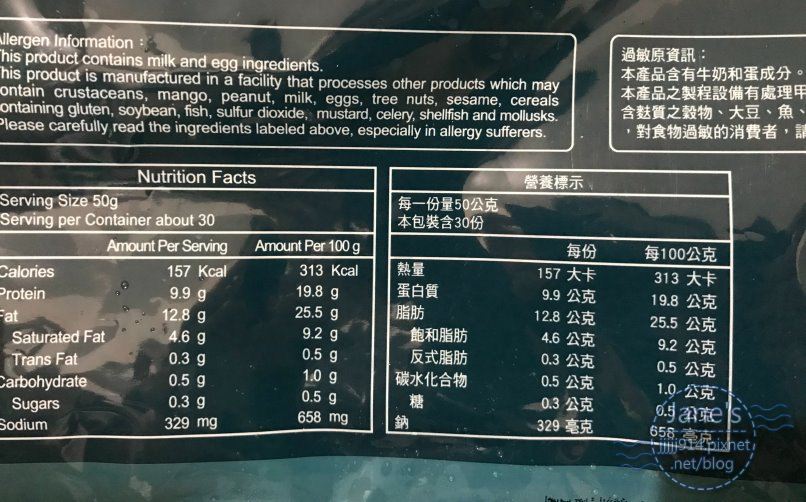The image displays a detailed ingredient list and nutritional information for a product, presented in both English and an Asian language, possibly Japanese or Chinese. The background features a gradient of black, gray, and greenish hues with a blurred reflection, while the text is outlined prominently in white font on a blue, non-solid background with indistinguishable images. At the top, a white-bordered rectangular section titled "Allergen Information" states that the product contains milk and egg ingredients and is manufactured in a facility that processes various other allergens, including crustaceans, mango, peanut, milk, eggs, tree nuts, sesame, cereals containing gluten, soybean, fish, sulfur dioxide, mustard, celery, shellfish, and mollusks. It advises carefully reading the labeled ingredients, especially for allergy sufferers.

Below the allergen information, there are multiple sections of text, some of which are written in Asian characters. The bottom left corner contains the nutrition facts, specifying a serving size of 50 grams with approximately 30 servings per container. The nutritional values per serving and per 100 grams are as follows: 157 kcal and 313 kcal for calories, 9.9 g and 18.8 g for protein, 12.8 g and 25.5 g for fat, 4.6 g and 9.2 g for saturated fat, 0.3 g and 0.5 g for trans fat, 0.5 g and 1.0 g for carbohydrates, 0.3 g and 0.5 g for sugar, and 329 mg and 658 mg for sodium, respectively. These nutritional details are similarly translated into the Asian language and presented in a corresponding box to the right. The bottom right corner features a logo with the text "Jane's n914.pixnet.net/blog."